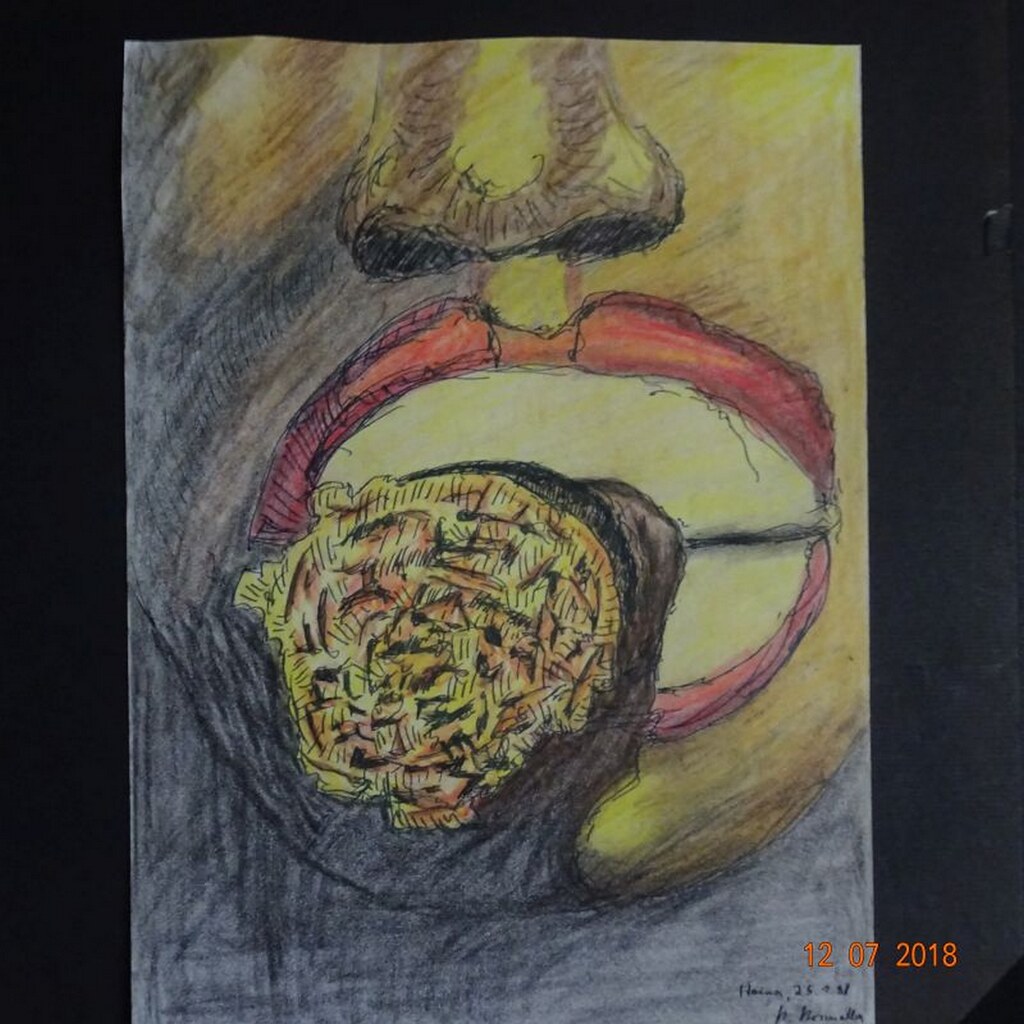This detailed colored pencil drawing, dated December 7, 2018, appears on an 8 by 11-inch sheet of loose white copy paper. The artwork portrays a partial face, meticulously capturing half of the nose, part of the cheek, the lips, and chin. A prominent feature in the drawing is a lit cigarette held between the lips. The tip of the cigarette is detailed with vibrant orange and yellow hues, indicating it is burning, and there are shades of gray suggesting smoke. The artist's use of color and shading brings lifelike detail to this expressive fragment of a human visage.